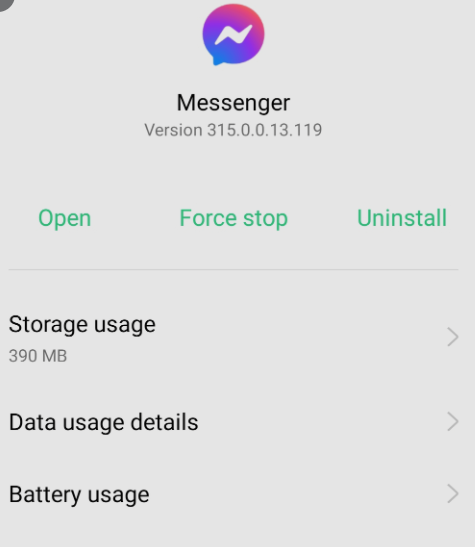The image is a partial screenshot displaying the settings section of a mobile device, specifically focused on the settings for the Messenger app. In the screenshot, the Messenger icon, a blue and purple speech bubble with a white lightning bolt inside, is prominently displayed against a gray background. Below the icon, black text indicates the app version as "Messenger version 315.0.0.13.119."

The editable options in the app settings are presented in light green text, offering three possible actions: "Open," "Force Stop," or "Uninstall." Further detailed options are listed below, providing additional information and navigational choices. For instance, the app is using 390 megabytes of storage, indicated next to a right-pointing arrow which suggests tapping it for more storage details. Similarly, data usage and battery usage details are also accessible via right-pointing arrows, inviting the user to delve deeper into those specific settings.